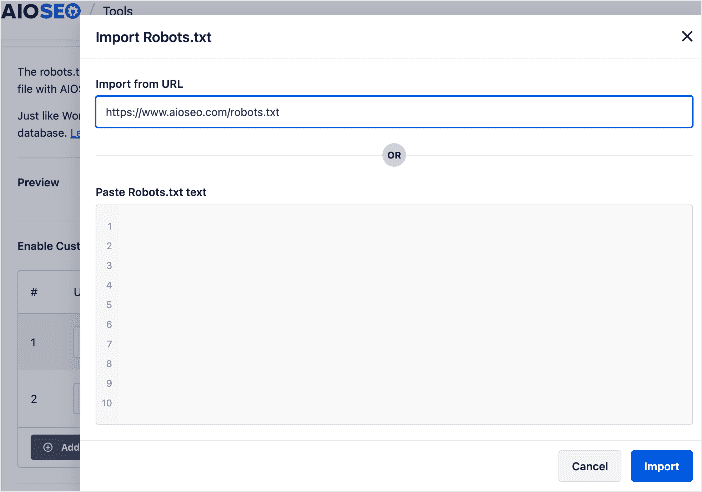The screenshot depicts a web interface of the AIOSEO plugin, specifically under the Tools section. The primary focus is a prominent white pop-up box titled "Import Robots.txt" located at the center of the screen, slightly obscuring the grayed-out background. 

In the top right corner of the pop-up, there is a conspicuous black "X" for closing the dialog box. Below the title, the interface offers two options for importing the robots.txt file. The first option allows users to enter a URL into a provided text field, pre-filled with the example "https://www.aioseocom/robots.txt." 

Alternatively, users may opt to paste the robots.txt content directly into a spacious gray rectangle, clearly labeled for this purpose. This text area is divided into ten distinct lines, numerically labeled from 1 to 10, each ready to accept inputted text.

At the bottom right corner of the pop-up, users are presented with two buttons: a white "Cancel" button and a blue "Import" button, offering clear options for proceeding or aborting the import process.